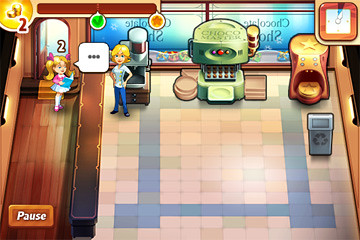The image is a screenshot from a video game rendered in a simplistic, non-photorealistic, artistic style. The perspective is a top-down, cross-sectional view of a room. The floor of the room is a dusty pink color, with a square drawn on it that contrasts with gray tiles. 

To the left of this main area, there is another room with a hardwood floor. Within this room stands a small cartoon figure—appearing to be a little girl with pale white skin and blonde hair tied in a ponytail. 

In the larger room, separated by a wall, there is another character that appears to be a boy, also with pale white skin and short yellow hair. The boy is dressed in a blue shirt and blue pants, standing against the simplistic, vibrant backdrop of the game.